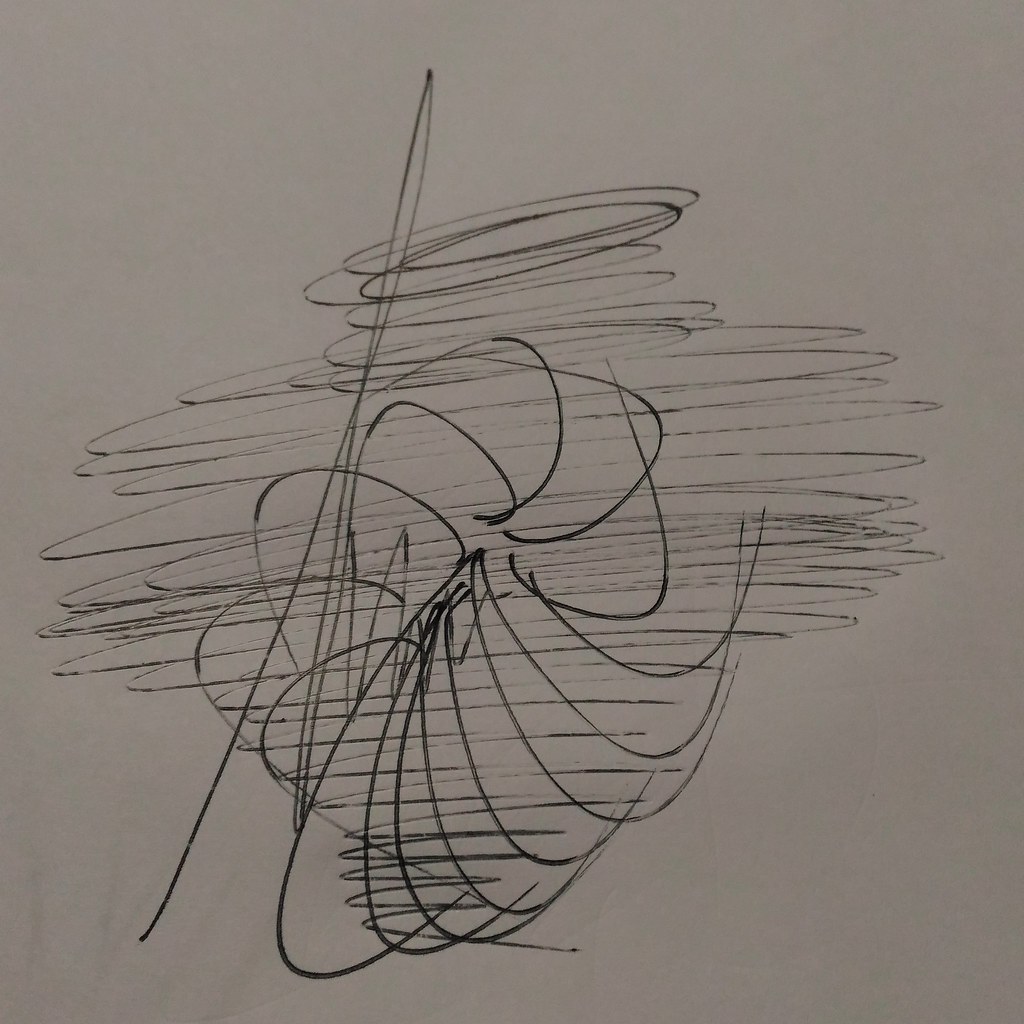This image showcases an abstract scribble drawing on a pale gray surface, likely a dry erase board. Traces of mostly erased previous scribbles are faintly visible, adding to the textured background. The central focus of the drawing is a continuous, cylindrical-shaped swirl of black, thinly drawn lines. These lines create a jug-like form through their back-and-forth motion, resembling a loosely constructed vortex.

Overlaying this primary shape is a more defined, darker set of lines that form a straight vertical line cutting through the middle of the jug shape. This line then transitions into a series of swirling patterns, reminiscent of a seashell or an anemone, adding depth and complexity to the composition. The two distinct shapes—the jug and the anemone-like swirl—intersect and interplay, creating a layered, intricate visual effect. The line work is crisp and clean, without any noticeable smudging, emphasizing the careful execution of the abstract forms.